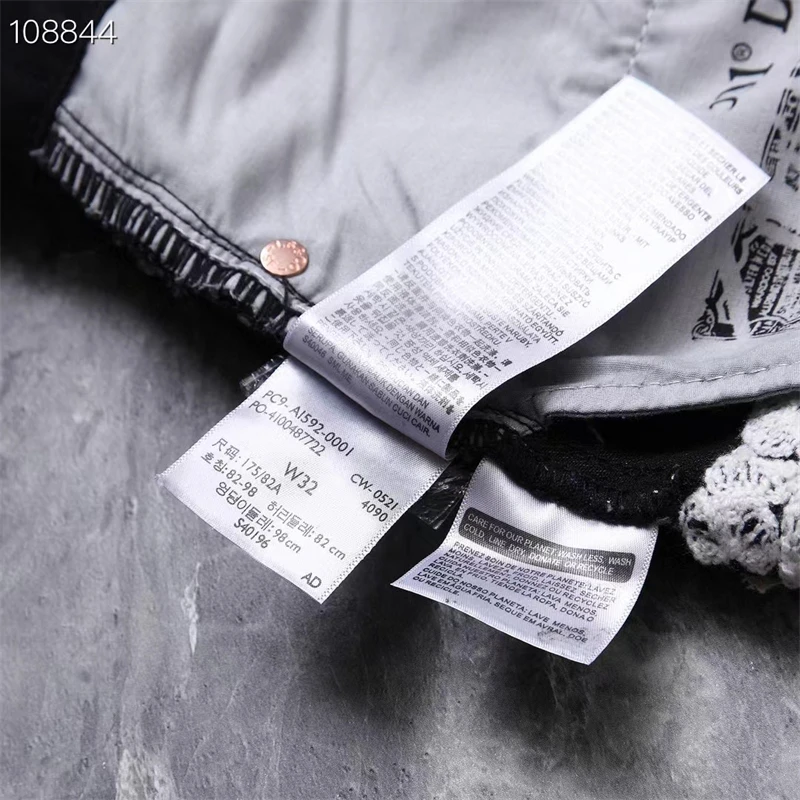This is a close-up shot of the inside of a pair of blue jeans, turned inside out to reveal the details of the tags and stitching. The white fabric of the pocket displays black text that reads "501." The garment features multiple tags: a white main tag with faint blue ink from washing, which indicates a waist size of W32 and includes Chinese characters; a longer tag situated above it with washing instructions in various languages; and a smaller tag to the right. Additionally, there are numbers, possibly the product number, 108844 and PC9A1592-001PO4100487722, visible on the tags. The jeans have gold grommets on the pocket and a gold button. The rough gray-black background contrasts with the blue fabric, enhancing the visibility of these details.